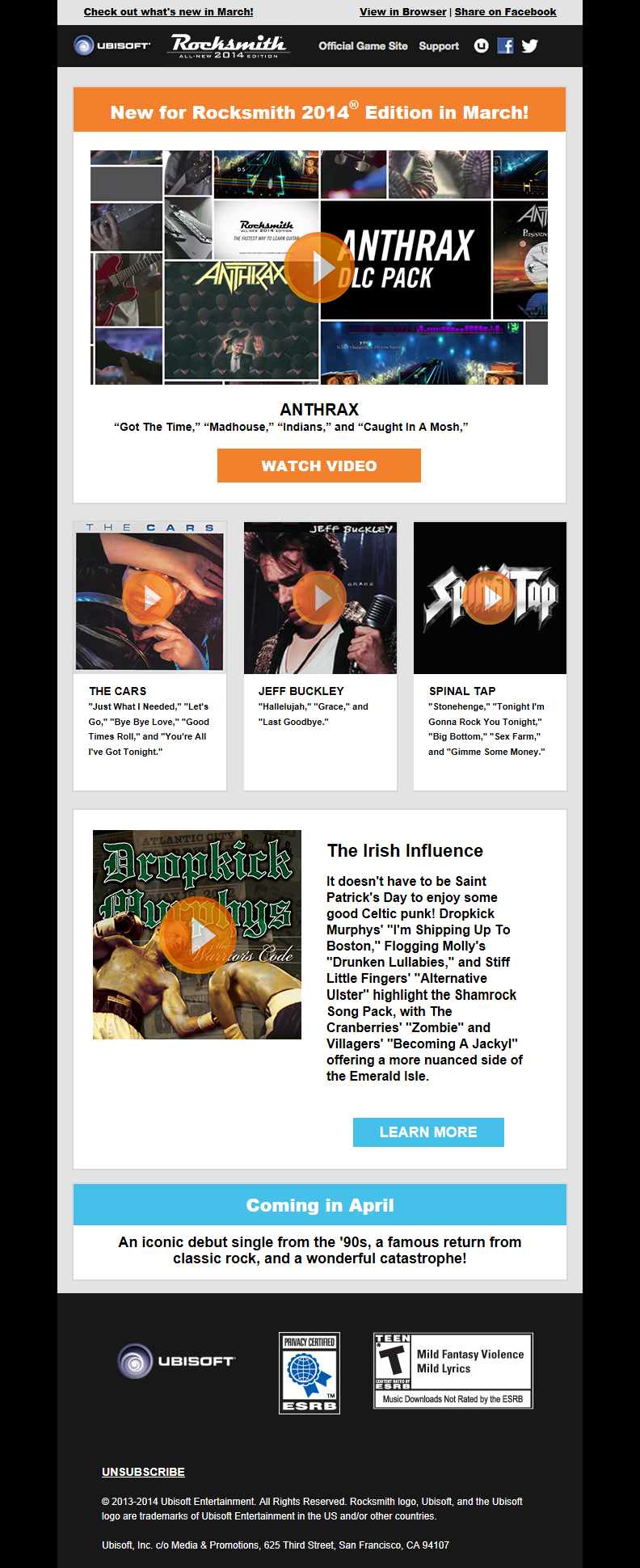This detailed caption provides an informative breakdown of the elements displayed in an image likely from an email or mobile webpage related to Ubisoft's Rocksmith 2014 edition:

---

This image is a promotional screenshot for Ubisoft's Rocksmith: All-New 2014 Edition from what appears to be a mobile device. At the top, there are options to “Check out what’s new in March,” “View in browser,” and “Share on Facebook.” Below this bar, the interface displays "Ubisoft, Rocksmith, Official Game Site Support" with three icons that likely link to Ubisoft's website, Facebook, and Twitter respectively.

The main section highlights new content available for Rocksmith 2014 in March. It features an Anthrax pack that includes the songs "Got the Time," "Madhouse," "Indians," and "Caught in a Mosh." Additionally, there's a Cars pack with the tracks "Just What I Needed," "Let's Go," "Bye Bye Love," "Good Times Roll," and "You're All I've Got."

Next, Jeff Buckley's featured songs "Hallelujah," "Grace," and "Last Goodbye" are listed. To the right, the screenshot showcases a Spinal Tap pack including "Stonehenge," "Tonight I’m Gonna Rock You Tonight," "Big Bottom," "Sex Farm," and "Gimme Some Money."

Toward the bottom, an article discusses the Irish influence in music, highlighting different groups and songs featured in the game that are from Ireland, performed by Irish bands, or have an Irish cultural influence.

The image gives the impression of being either a webpage or an email due to the inclusion of an unsubscribe link at the bottom, a common feature in email communications.

---